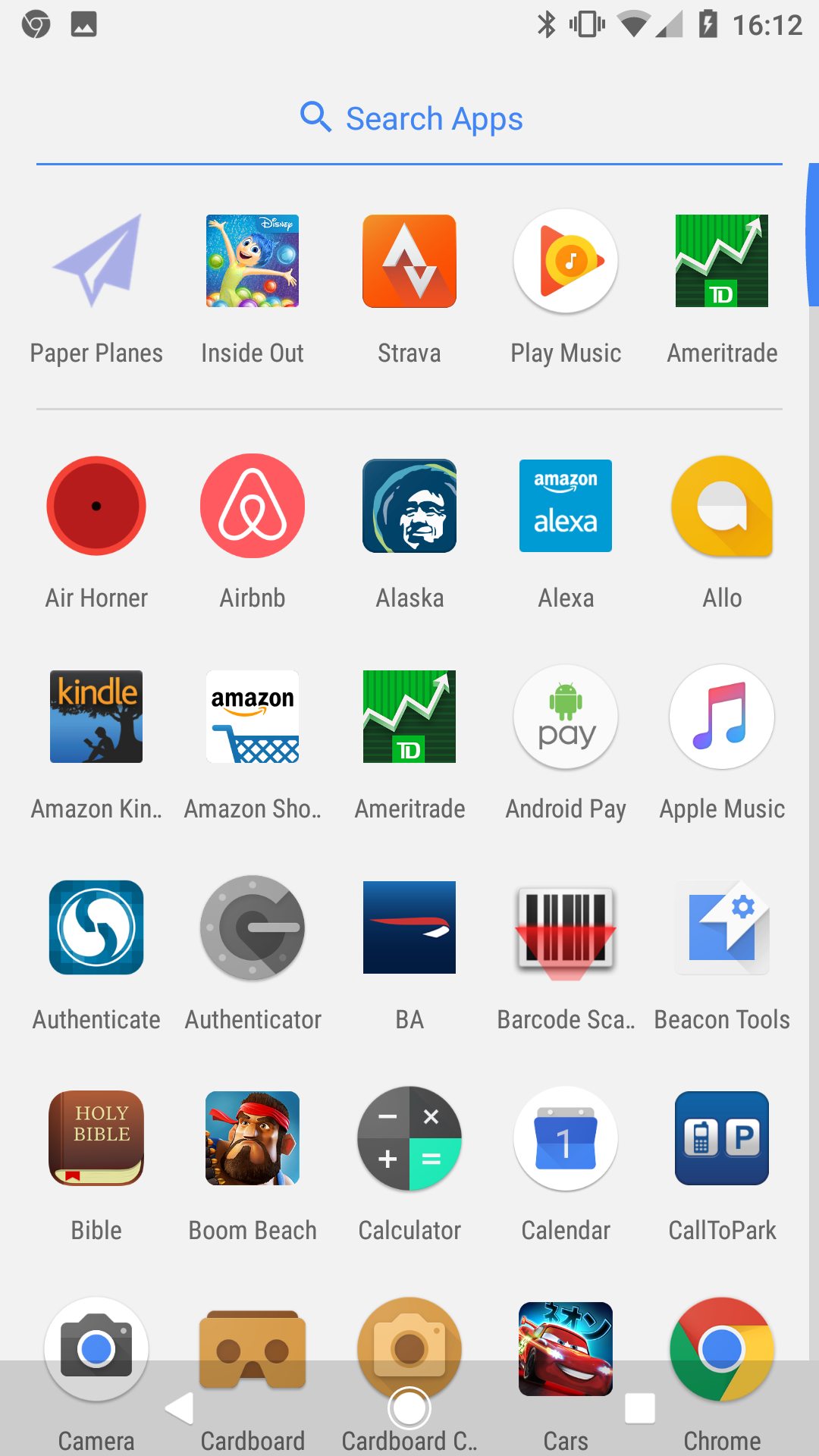This is a screenshot of an Android mobile device showcasing its application search feature. The screen, set against a gray background, displays a search bar at the top below the status bar, with the prompt "search apps" next to a magnifying glass icon in blue text. The layout includes six rows of application icons, each row containing five colorful icons. Prominently featured are the five most recently searched or used apps: Paper Planes, Inside Out, Strava, Play Music, and Ameritrade. Following these is the complete alphabetical list of applications installed on the device, beginning with Air Horner. The final app visible in the bottom right corner of the screen is Chrome.